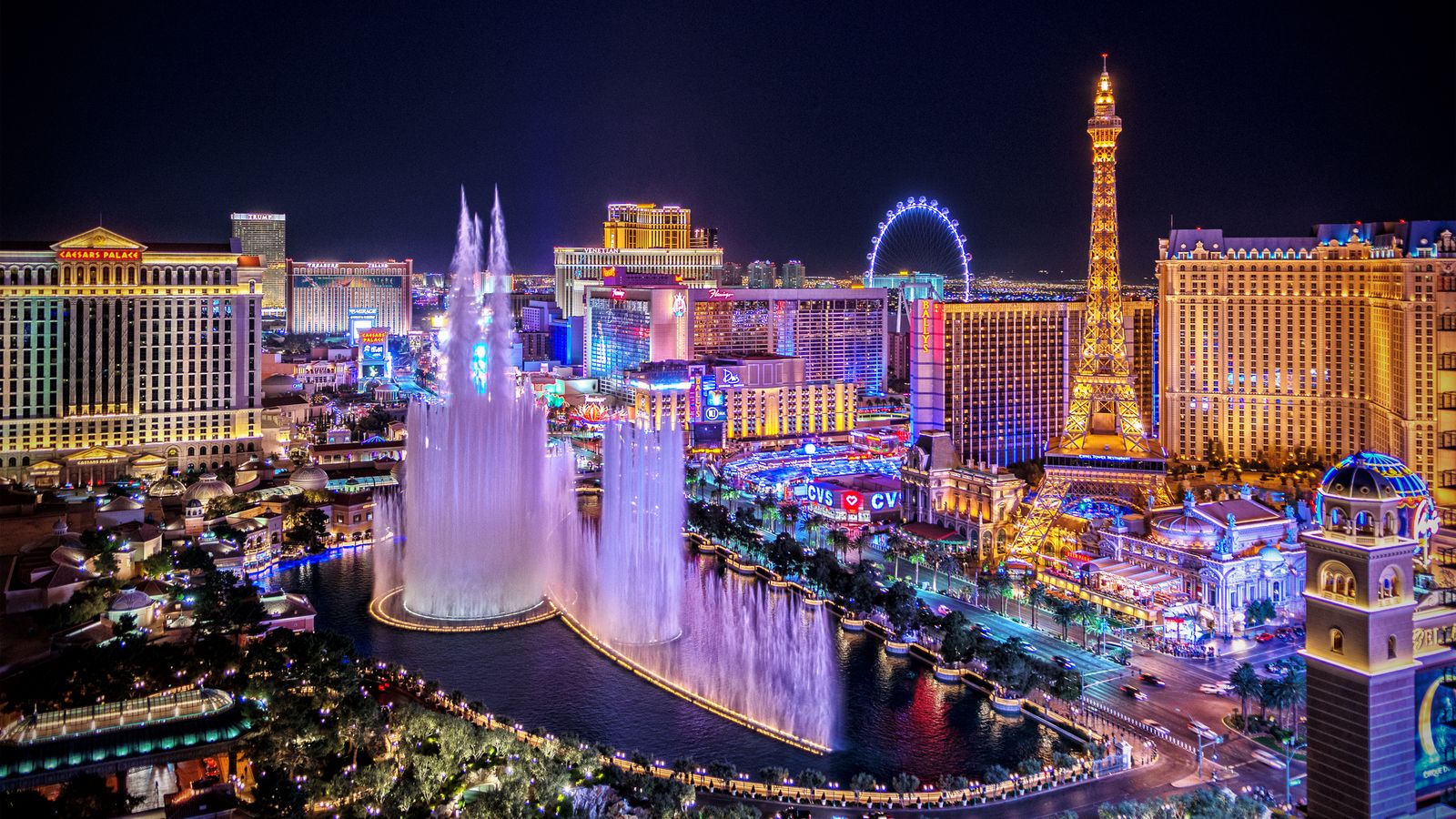The nighttime image captures a vibrant cityscape, unmistakably Las Vegas, vividly illuminated by a spectrum of neon colors. Dominating the right side of the frame is the replica of the Eiffel Tower, surrounded by various buildings adorned with glowing blue and neon lights. In the center lies a grand, man-made body of water featuring spectacular fountains whose water jets soar impressively high, higher than many of the surrounding hotels. These fountains are likely those of Caesars Palace, identified by its distinct red signage to the left of the picture. A lit-up Ferris wheel is visible in the background, casting hues of blue, pink, and gold across the scene. Numerous other brightly lit hotels and casinos form the backdrop, including a notable CVS pharmacy nestled close to the fountains. The image presents an aerial view of this bustling, colorful city, emphasizing its lively, almost surreal ambiance reminiscent of an illuminated wonderland.